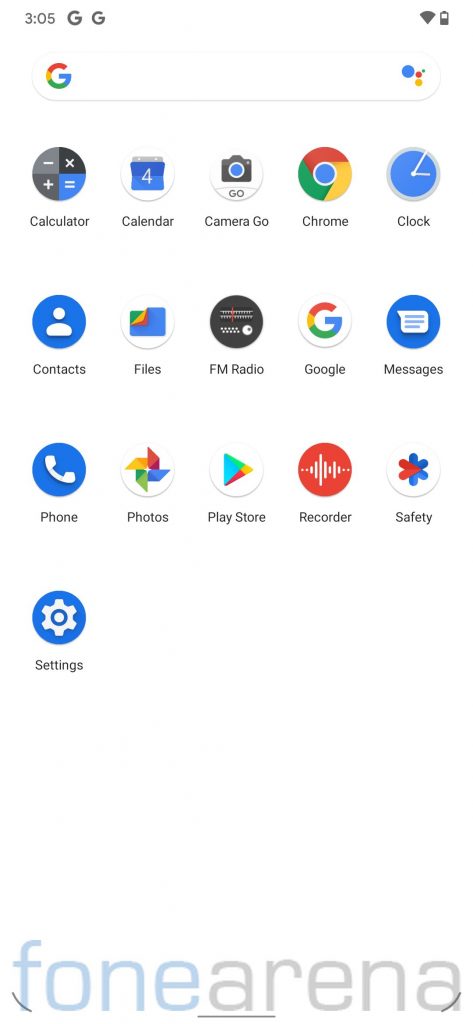This is a detailed caption for the provided image:

---

This is a screenshot from a smartphone displaying its home screen filled with various app icons and options. At the bottom of the screen, a horizontal banner reads "PhoneArena," though "Phone" is misspelled as "Fone." The top of the screen indicates the time as 3:05 and features two Google icons. A prominent Google search bar is positioned beneath the time display. Below the search bar, there are four rows of app icons. The first three rows each contain five icons, while the fourth row contains only one icon. These icons are organized horizontally across the screen and include: Calculator, Calendar, Camera Go, Chrome, Clock, Contacts, Files, FM Radio, Google, Messages, Phone, Photos, Google Play Store, Recorder, Safety, and Settings. In the upper right-hand corner, a Wi-Fi icon is visible alongside a battery icon showing a half charge.

---